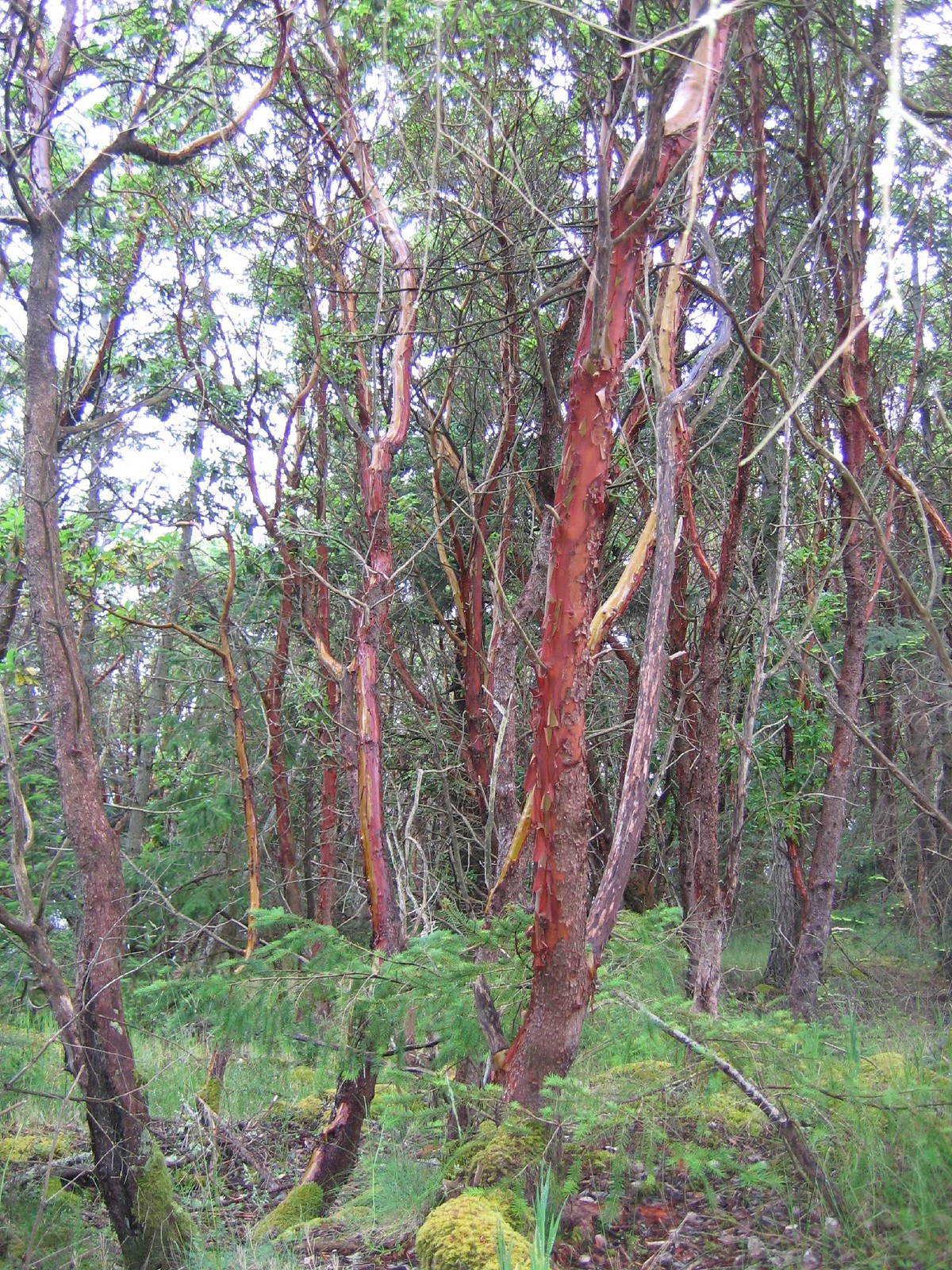In this professionally taken photograph of a wooded forest, numerous trees dominate the scene. Prominently, some of these trees exhibit vibrant reddish-brown trunks, with bark that is peeling to reveal layers of red and even greenish hues underneath. Additionally, numerous healthy trees, covered in typical brown bark and green leaves or pine needles, contribute to the rich tapestry of this forest environment. The foreground is carpeted with patches of moss, yellowish-green and red plants, stones, and rocks interspersed among high, green grasses. Through the canopy of branches—some bare, some lush with foliage—a sky of pale white and hints of blue is visible, creating a glare that suggests bright sunlight filtering through.